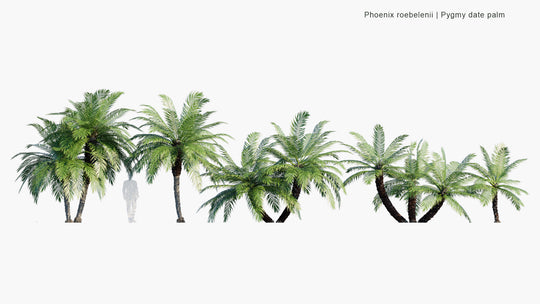The image showcases five beautifully illustrated pygmy date palm trees, scientifically labeled as "Phoenix Robaenae Pygmy Date Palm" in small text located at the upper right corner. Each palm tree exhibits lush green fronds and sturdy, dark brown trunks, though their bases are not visible. The trees are distinct in their arrangement, some forming pairs while others stand alone. Situated between the first and second palm tree on the left, there's a gray silhouette of a man dressed in white, hands in his pockets, serving as a scale reference to emphasize the trees' height. The entire setting is minimalistic and modern, with neutral, muted colors and a clear, detailed lighting that accentuates the contemporary style of the illustration, which is presented in a landscape format.